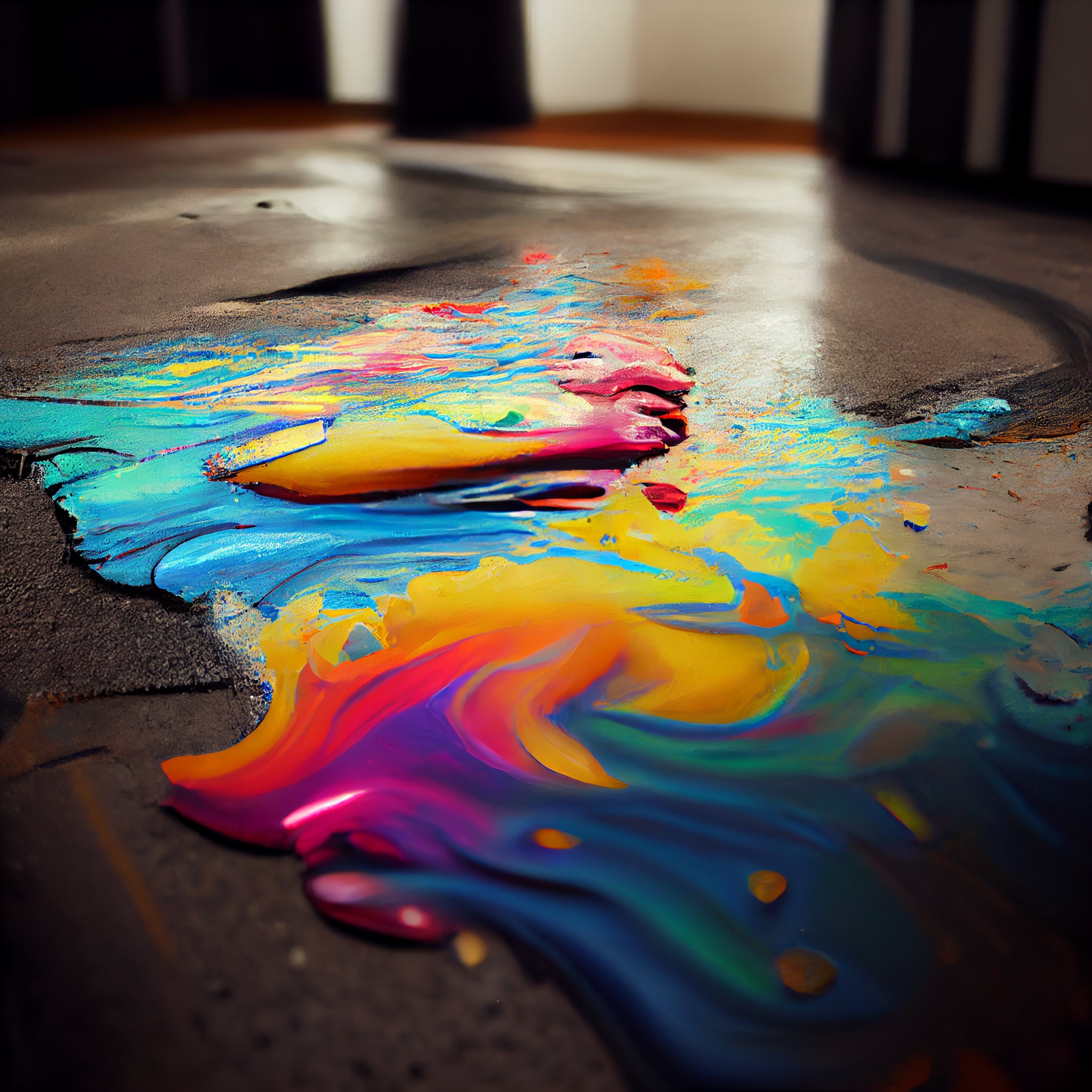The photograph captures the abstract art created by the spillage of thick acrylic paint on an uneven, brownish or rust-colored floor, which features visible cracks and lines. The predominant colors in the artwork are blue, orange, and yellow, mixed with hints of pink, purple, and green, forming wave-like, floral, and swirl patterns that appear almost three-dimensional. The background is slightly blurred, showing white walls with wood trim and some darker sections. The overall aesthetic is a striking blend of accidental and purposeful paint application, evoking a sense of spontaneous yet deliberate creativity.